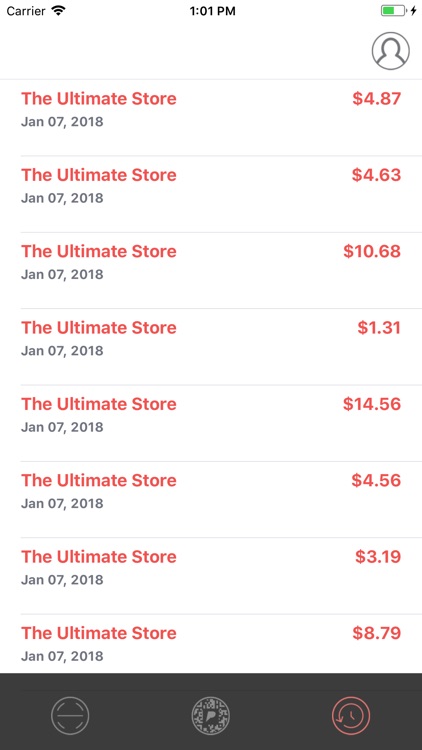### Descriptive Caption:

A detailed screenshot depicting a bank statement viewed on a mobile device. The device clock shows 1:01 PM, and the battery icon, currently at approximately 50%, indicates it is being charged. The network signal is visible alongside the carrier name. 

The screen primarily displays a silhouette profile icon at the top, followed by a list of eight transaction entries, all from "The Ultimate Store" and dated January 7th, 2018. Each entry shows the transaction amount in red and the date in black, arranged in descending order:

1. $4.87
2. $4.63
3. $10.68
4. $1.31
5. $14.56
6. $4.56
7. $3.19
8. $8.79

At the bottom of the screen, there is a prominent black "R" symbol, accompanied by a couple of circular icons featuring various white symbols, the specifics of which are unclear. This comprehensive screenshot provides a concise overview of the transaction history on that date.